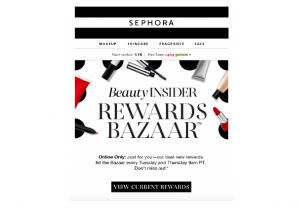This image from the brand Sephora is a compact, vertical layout featuring a series of structured sections. At the very top, a black horizontal bar spans the width of the image. Below this, a white section showcases the word "SEPHORA" in bold, black, all-capital letters. Following that is another black horizontal rectangular section.

Under these sections, four categories are listed horizontally, with the first visibly marked as "Makeup" while the other three remain unreadable due to the image's small size. In the center of the image, the word "BEAUTY" appears prominently, followed by "INSIDER" in bold, black, all-capital letters. Directly beneath this, the word "REWARDS" is displayed in a slightly larger font, maintaining the same bold, black, all-capital style, followed by "BAZAAR" on the next line.

"Online Only" appears below in bold, tiny, black font, accompanied by an unreadable phrase in unbolded, black font. The bottom of the image features another black horizontal rectangle containing white text.

Surrounding the central white background are various beauty items. Notably, there is a red lipstick with its cap off positioned in the middle of the right side. Slightly higher is a tan-colored item, possibly a small tube. At the top-center, what appears to be a mascara in a silver tube is displayed, along with other smaller beauty items scattered around.